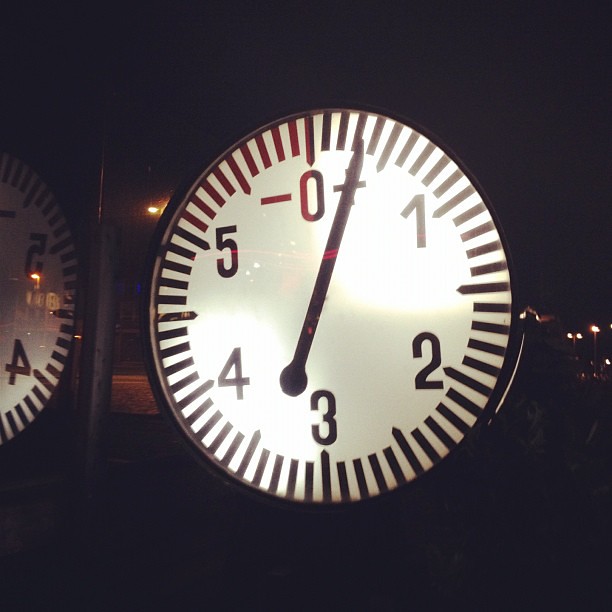The image depicts a close-up of a circular gauge resembling a clock face, set against a black background with faint light in the distance. The dial features numbers from 0 to 5, with intermediate markers, more prominent at every fifth increment. The gauge's single hand is positioned slightly above 0. To the left and right of the 0, there are minus and plus signs, respectively. The dial itself is white, while the entire photo foreground is nested against a darker setting, where another similar, slightly visible circle might be a reflection.